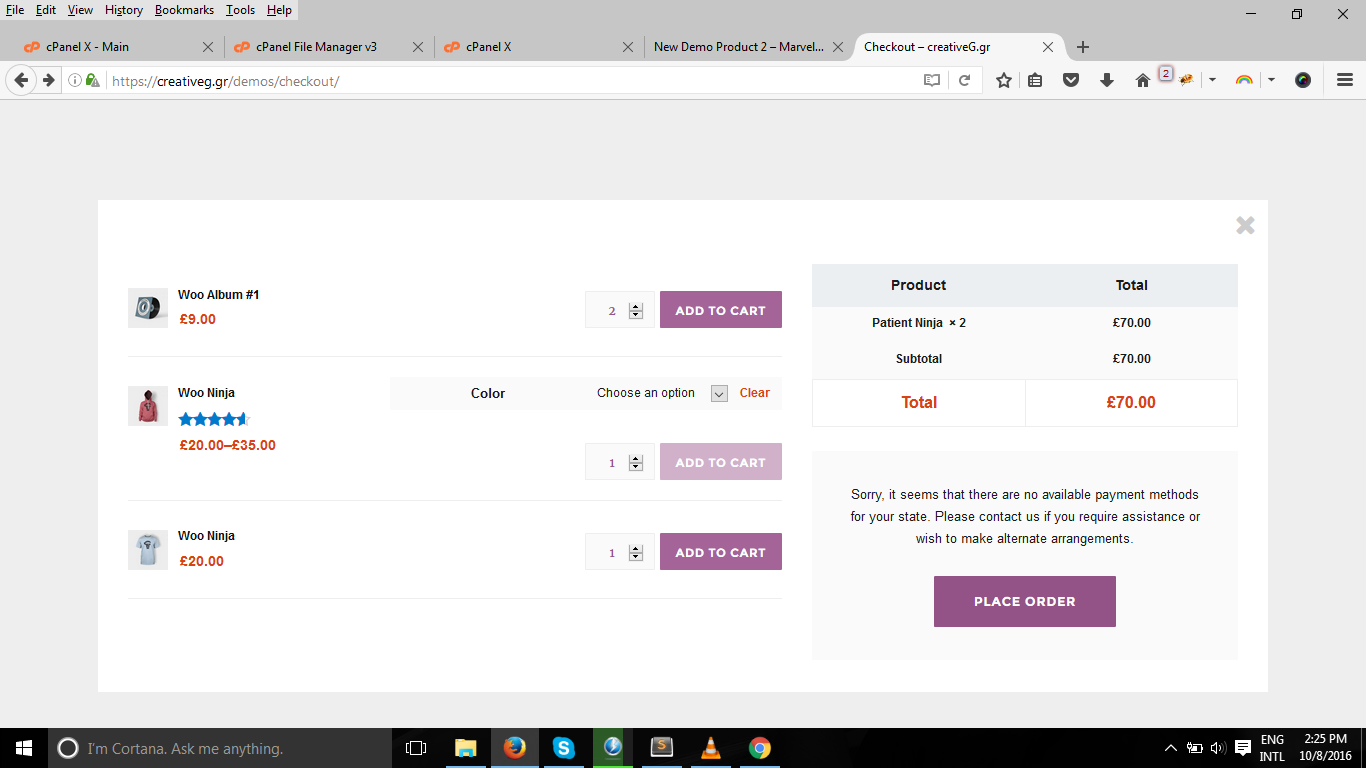This screenshot displays an open checkout page from a website, titled "Checkout - Creative.g.gr," with five browser tabs visible at the top. The shopping cart contains three items. The first item listed is "Woo Album #1," priced at £9 with the price highlighted in orange. The second item is "Woo Ninja," with a price range of £20-£35. The third item is another "Woo Ninja," identified as a t-shirt, priced at £20. The cart summary indicates a total of two "Patient Ninja" items, collectively priced at £70. Next to these items, there are optional add-ons available. At the bottom of the cart summary, there is a prominently displayed purple rectangular button labeled "Place Order."